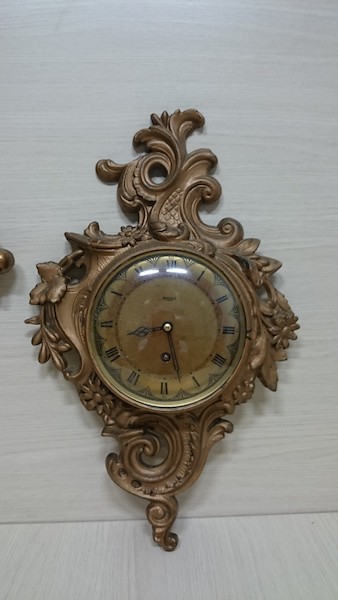The image depicts an ornate, antique-styled clock, likely crafted in a Baroque or Rococo design. The round dial of the clock features Roman numerals from I to XII in black, encased in a light brown or deep golden face. The clock is enclosed in a lavish bronze or brass-colored case adorned with intricate scrolls, swirls, and leaf motifs, which extend above and below the clock face, possibly serving as supports to stand it up. The surface behind the clock appears to be a painted white wood, with visible wood grain, suggesting it might be mounted on or resting against a paneled wall. The clock hands are also black and are currently set to approximately 8:27. The face of the clock is covered with glass that reflects overhead strip lights, adding to the vintage aesthetic of the piece.